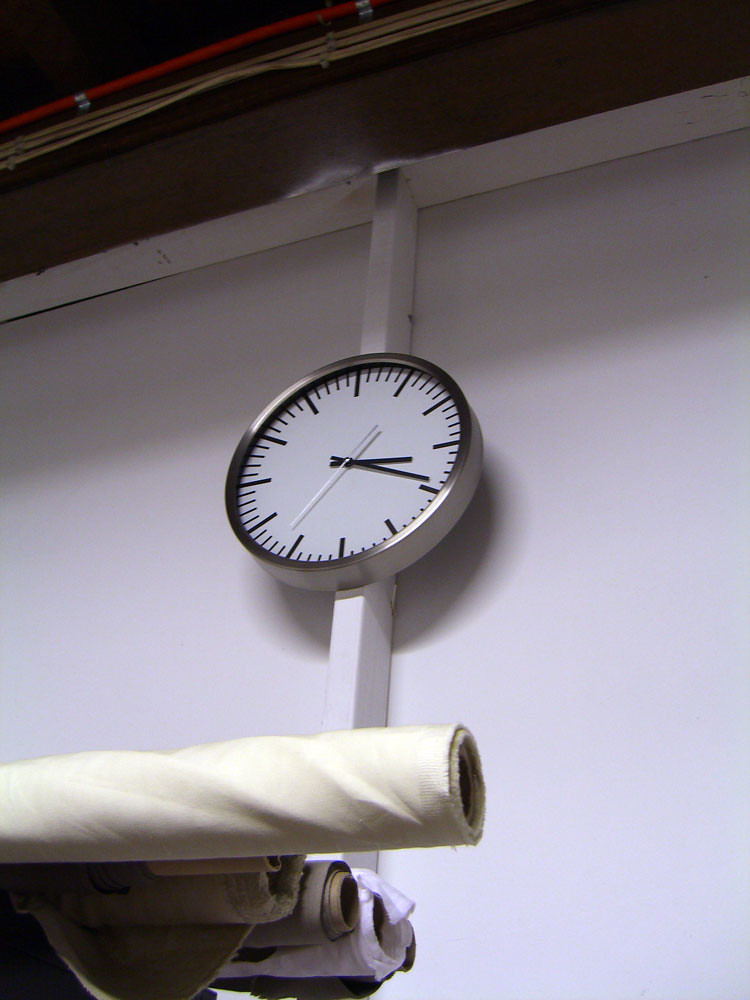The photograph captures a textile warehouse with a focus on a clock mounted on a vertical white post against a white wall. The clock, which features a shiny silver metal circular frame and a white interior, lacks numbers and instead uses black dash marks to indicate numerical positions. It has a black hour hand pointing towards the three, a black minute hand just before the four, and a clear or white second hand just past the seven. Below the clock in the bottom left-hand corner of the image, there are several rolls of fabric in shades of beige, white, and gray, wrapped around cardboard tubes. The top portion of the image reveals a darker metal ceiling with horizontally stretched, thin tan wires, and a thicker red wire. The clock is set to approximately 3:19.